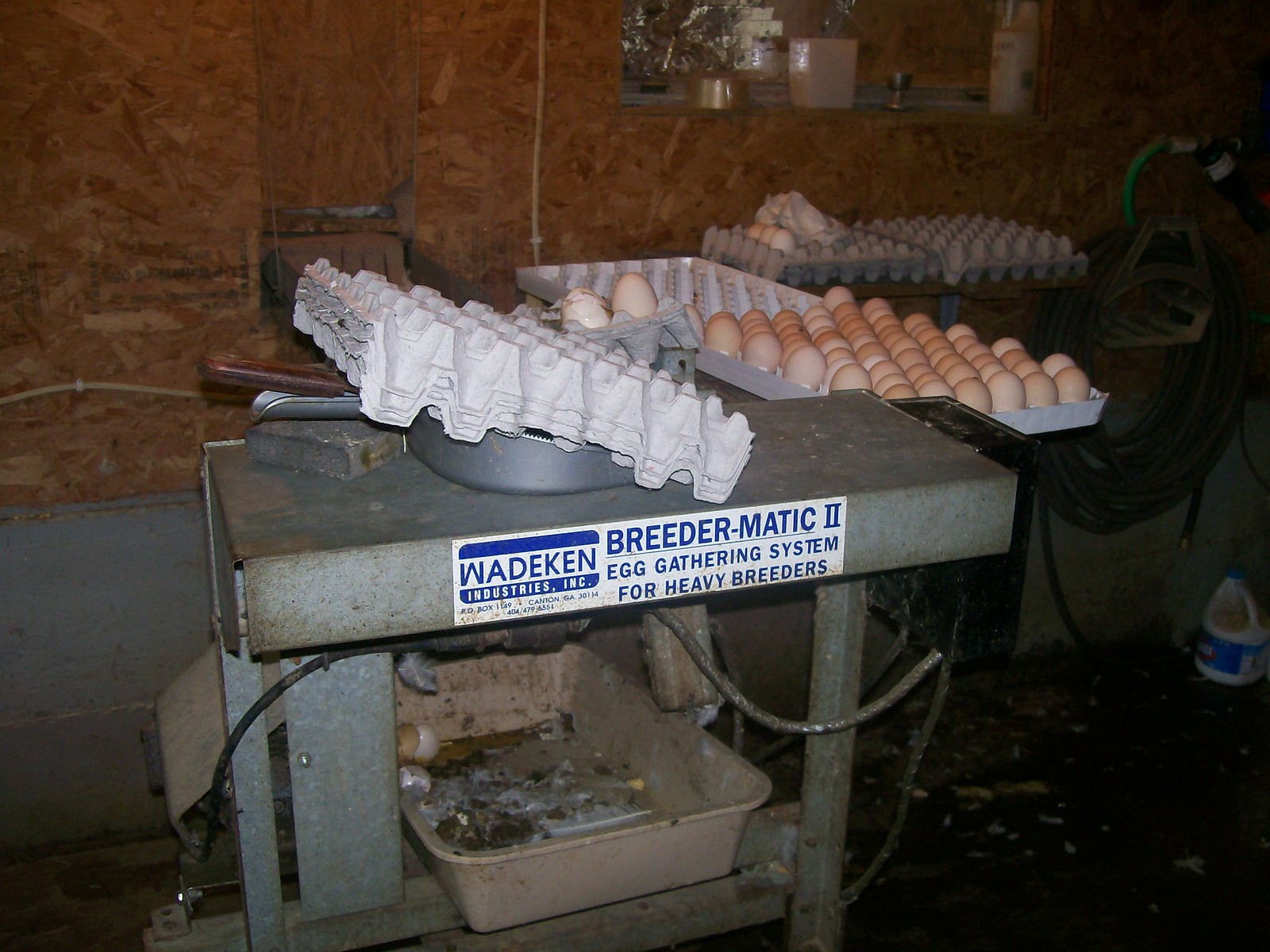The photograph depicts a Breedermatic 2 egg-gathering system by Wadeken Industries Inc. at the center. The machine is featured on a metal table, which holds large egg cartons. These cartons, designed for heavy breeders, contain different shades of brown eggs, some stacked and others filled, each holding dozens of eggs. A very large carton near the machine appears to hold about 50 eggs. The table has a white label with blue lettering indicating the machine’s manufacturer and model. Beneath the table lies a faded pink plastic tray, filled with feathers, eggshells, and dirt. The room is dimly lit, highlighting a plywood wall with a rope attached to a holder and a bottle of Clorox bleach to the right.